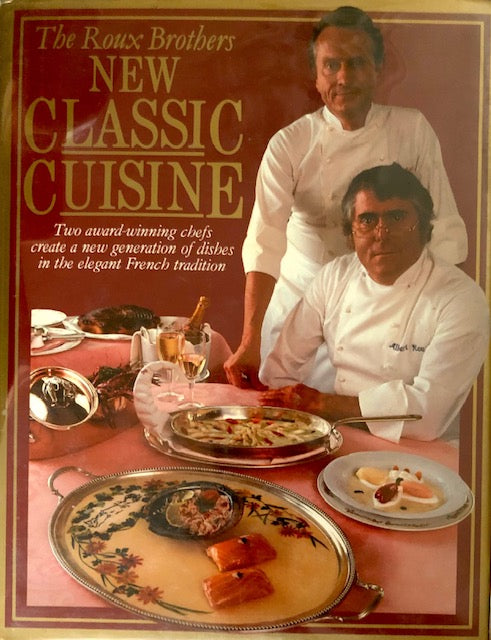This image features the cover of a cookbook titled "The Roux Brothers New Classic Cuisine," showcasing two men, presumably the Roux brothers, who are award-winning chefs specializing in elegant French cuisine. The two chefs are clad in white chef uniforms, with one seated and the other standing. The cover is primarily burgundy with gold lettering and trim, and additional text in a tan color. Below the title, it reads in white text: "Two award-winning chefs create a new generation of dishes in the elegant French tradition." In front of the chefs, an array of dishes is displayed, including platters with intricate arrangements, possibly featuring items such as flowers, what appears to be a salmon, a dish with sauce or gravy, and a large skillet that might contain a pasta dish. Additionally, there's a bottle of champagne in a chilling container with a towel in the background.